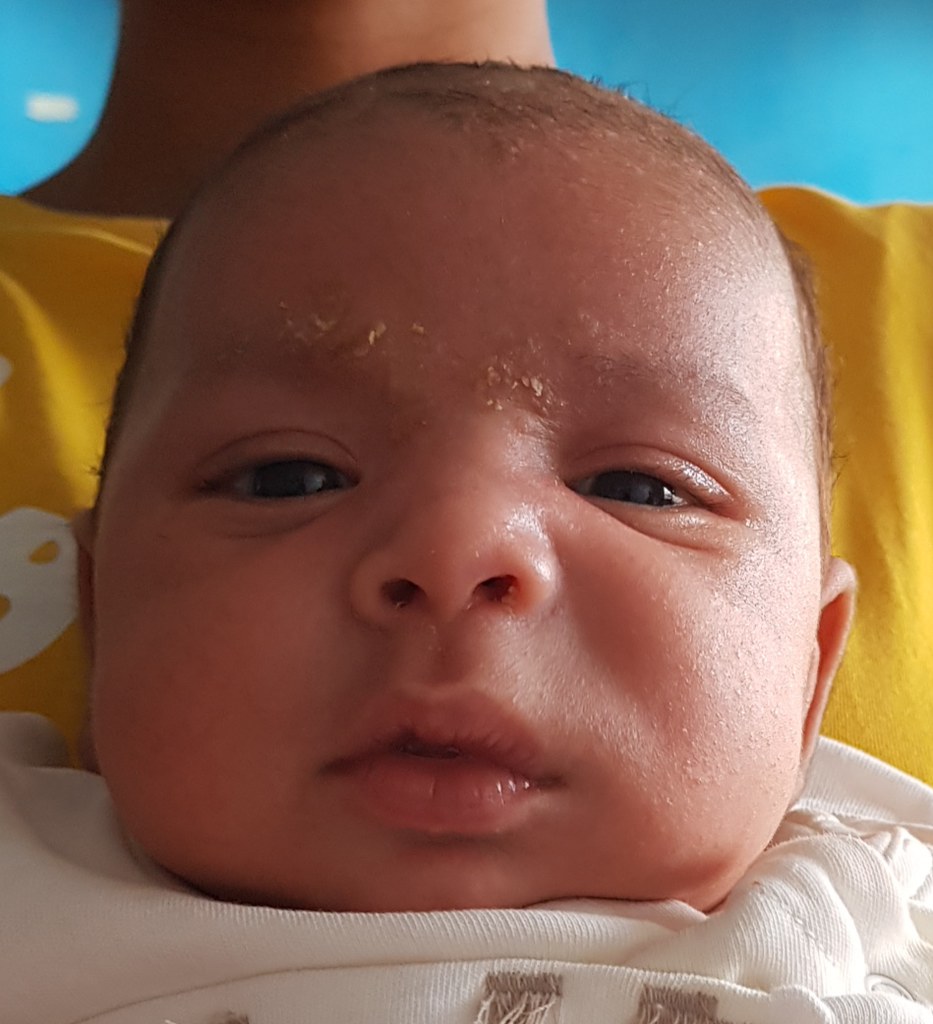This image is a very close-up shot of a newborn baby with pink skin and dark brown eyes that are barely open. The baby has slightly open lips and a noticeable patch of flaky skin or possibly cradle cap on its forehead between the eyebrows. A thin layer of fine, dark, possibly black hair covers its head. The baby is dressed in a white and brown outfit, resting on what appears to be someone's lap. The person holding the baby is wearing a yellow shirt, and while it is unclear if it is their leg or arm that appears in the top left of the image, a part of their neck is visible. The blue background with a small white cloud adds a soft touch to the scene. Despite a mention of peanut butter on the baby’s forehead from one of the descriptions, it seems more likely to be dry skin.